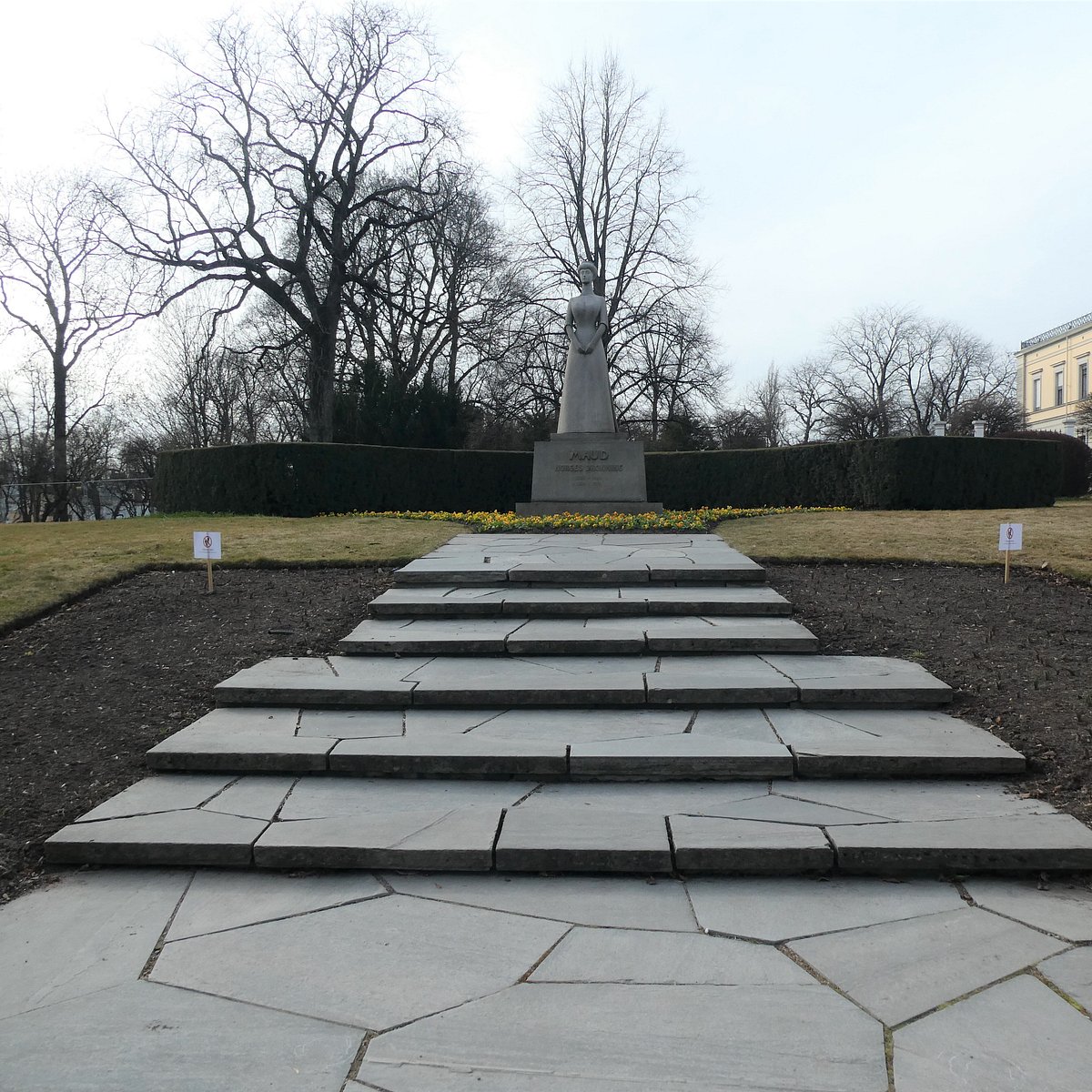The image features a detailed scene centered around a gray statue of a woman in a long gown, with her hands together in front of her. This statue is mounted on a square cement slab that has the name "MAUD" engraved at its base. The statue is surrounded by a well-trimmed, dark green hedge that forms a half-circle around it, creating a backdrop of neat symmetry.

Leading up to the statue are seven broad, shallow steps made from cut stone, designed with intricate patterns and intentionally fragmented to add a rustic charm. These gray stony stairways decrease in width towards the top, almost like small platforms. Along both sides of the stairway is dark soil with small green plants sprouting from it.

At the top of the steps, on either side, green and yellow grass forms a narrow lawn that expands into a flowerbed filled with tiny yellow flowers. These flowers seem to fan out around the base of the statue, complementing the well-trimmed hedge behind it.

On each side of the stairway, planted in the soil, are two wooden signs with white tops, standing firmly in the ground. The background reveals a landscape transitioning into autumn or winter, with a mix of trees—some still bearing green leaves while others are bare. To the right side of the image, a shade of yellow building peeks from behind the scene, and to the left, near the hedge, there appears to be a body of water. The sky above is an overcast white, completing the serene yet intricate portrayal of this peaceful setting.